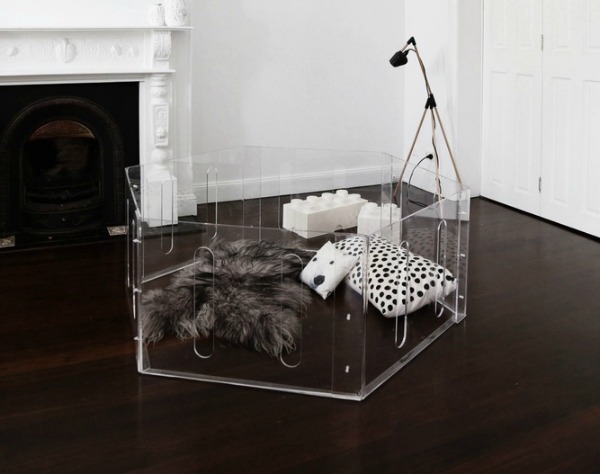In the midst of a modern, predominantly white living room, there stands a clear, acrylic enclosure reminiscent of a baby gate or playpen, suitable for pets or infants. This hexagonal structure resides centrally on a dark brown wooden floor. Inside the enclosure, there is a black and white furry cushion, a white pillow adorned with a dog face, and another larger white pillow with black polka dots. To the right of the enclosure, there is a distinct dog-themed pillow and a longer white pillow with polka dots. Adjacent to the enclosure, large, white, rectangular Lego blocks add a playful element to the room. In the background, a white fireplace with a black front and a small black door adds a touch of coziness. A white double door is visible on the right, while a plugged-in tripod lamp stands nearby, illuminating the scene.